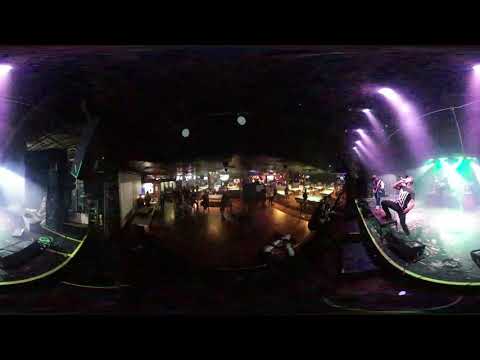The image captures a live concert in an indoor nightclub with a dimly lit atmosphere. The foreground features a stage on the right-hand side, illuminated by vibrant pink, purple, blue, and green spotlights. On stage, a singer, holding a microphone close to his mouth and standing with one foot on a speaker, performs energetically. Beside him, a guitarist plays, perhaps near the dimly visible drummer bathed in blue light. The stage's front has a distinctive yellow trim. Central to the venue, there's a wraparound bar area with a few patrons seated. The seating is sparse, with only a handful of viewers scattered around the tables and in front of the stage. The floor is wooden, contributing to a bar-like ambiance, and towards the back, one can spot pool tables, suggesting this is a multipurpose bar or activity venue. Interestingly, a mirrored or possibly a 360-degree stitched image effect shows what seems like an identical stage on the left, adding a warped, curvilinear feel to the photograph.